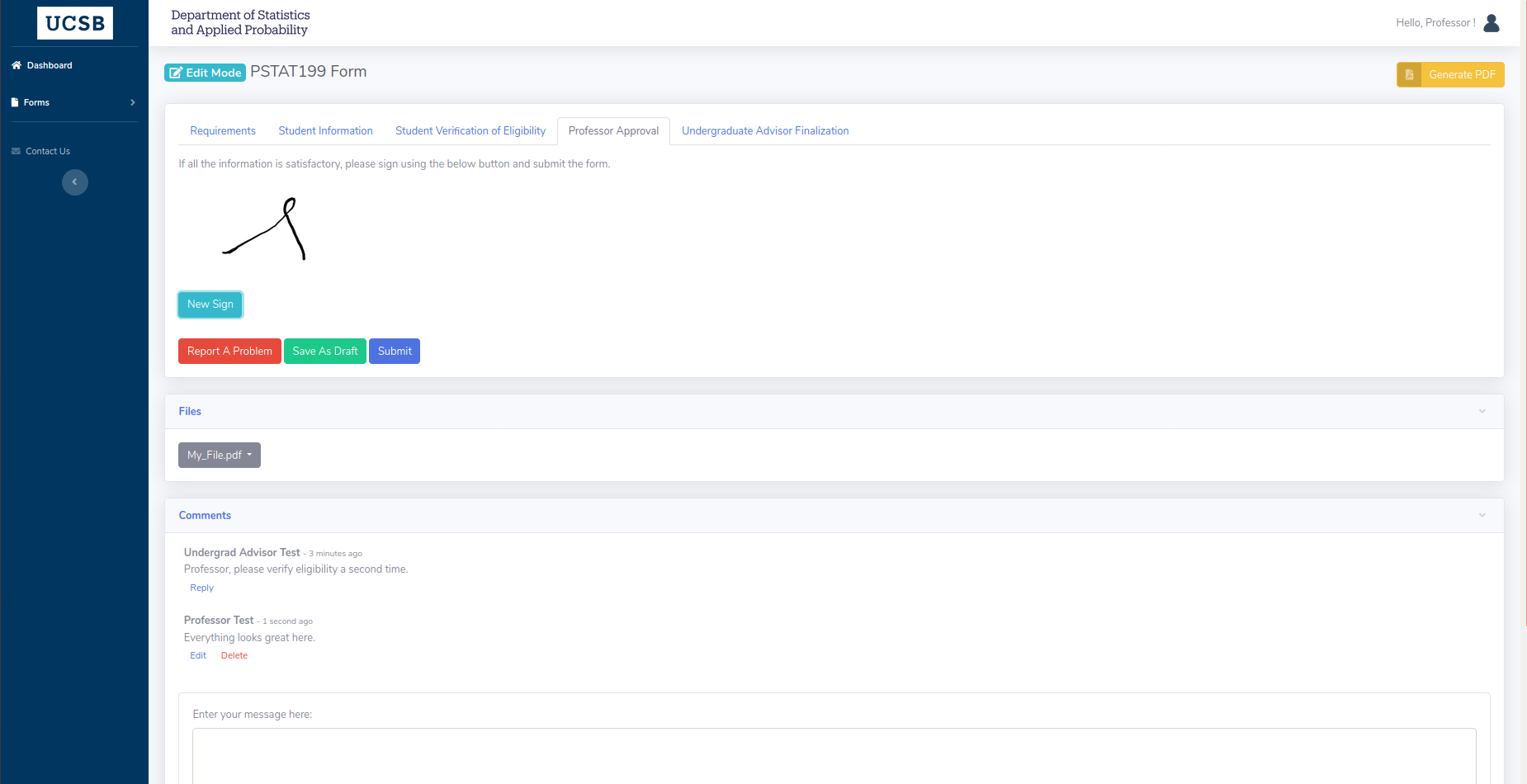The image appears to be a screenshot of a computer or laptop monitor showing an application or web interface. On the left side, there is a vertical rectangle filled with a dark blue color. At the top of this blue section, within a horizontal white-filled rectangle, the text "UCSB" is displayed in black letters. Below "UCSB," there are menu options labeled "Dashboard," "Forms," and "Contact Us."

To the right of the blue section, the header reads "Department of Statistics and Applied Probability" in black letters. Just below this header, the words "Edit Mode" and "PSAT 199 form" are visible. The content of the form includes several sections labeled "Requirements," "Student Information," "Student Verification," "Availability," "Professor Approval," and "Undergraduate Advisor Finalization."

A paragraph of black text under these sections instructs: "If all the information is satisfactory, please sign using the below button and submit the form." Following this instruction is a line indicating a signature space labeled "New Sign."

At the bottom of the form, there are three buttons labeled "Report Problems," "Save Draft," and "Submit." Further down, a section labeled "Files" is shown, with an attachment named "myfile.pdf." Beneath the file attachment area, there is a section for comments.